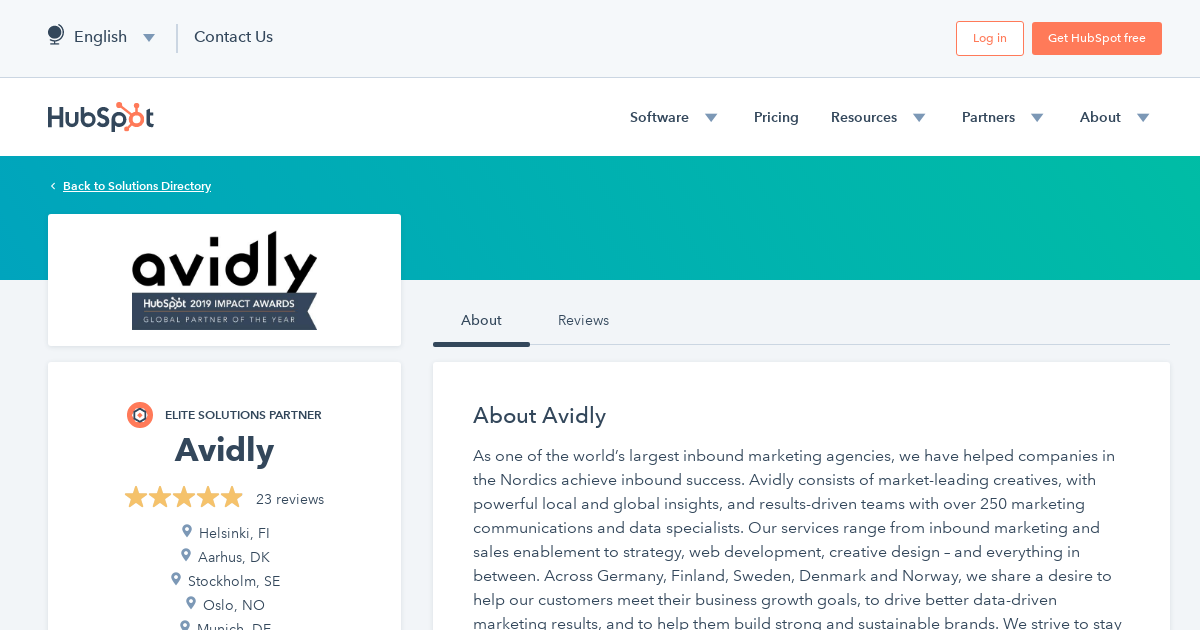**Detailed Caption for Informational Website Screenshot:**

The screenshot captures an informational page from a website. At the top left corner, there is a light gray header featuring a dark gray globe icon followed by the text "English" in dark gray and a gray arrow pointing down. This is separated by a thin vertical gray line from the adjacent text "Contact Us" in dark gray, with significant negative space extending to the right of it. 

In the top right corner, two buttons are visible: a white button with an orange outline and orange text that says "Login," and a wider orange button with white text that reads "Get HubSpot Free."

Underneath the top header, a medium gray thin line delineates it from the subsequent header, which is white. On the left side of this white header, "HubSpot" is written in gray text with the "O" in orange, adorned with three node-like objects branching off. To the right, there are dropdown menus and sections in gray text labeled "Software" with a gray arrow pointing down, "Pricing," "Resources" with another gray arrow, "Partners" with another gray arrow, and "About" with yet another gray arrow.

Below this header, there's a color gradient banner transitioning from teal blue on the left to aqua blue on the right. At the top left of this gradient banner, white underlined text reads "Back to Solutions Directory," accompanied by a left-pointing arrow. Overlaid on the left side of this gradient background is a prominent white rectangle featuring the word "Avidly" in black text at the top center. Below this, a gray banner icon appears with "HubSpot 2019 Impact Awards" written in white text and underlined in red. Beneath this, smaller white text reads "Global Partnership of the Year."

Lastly, under this gradient header, a white sidebar is situated on the left, leading to the main body of the page on the right. The main body is characterized by a light gray background with a central white rectangle containing a substantial amount of text.